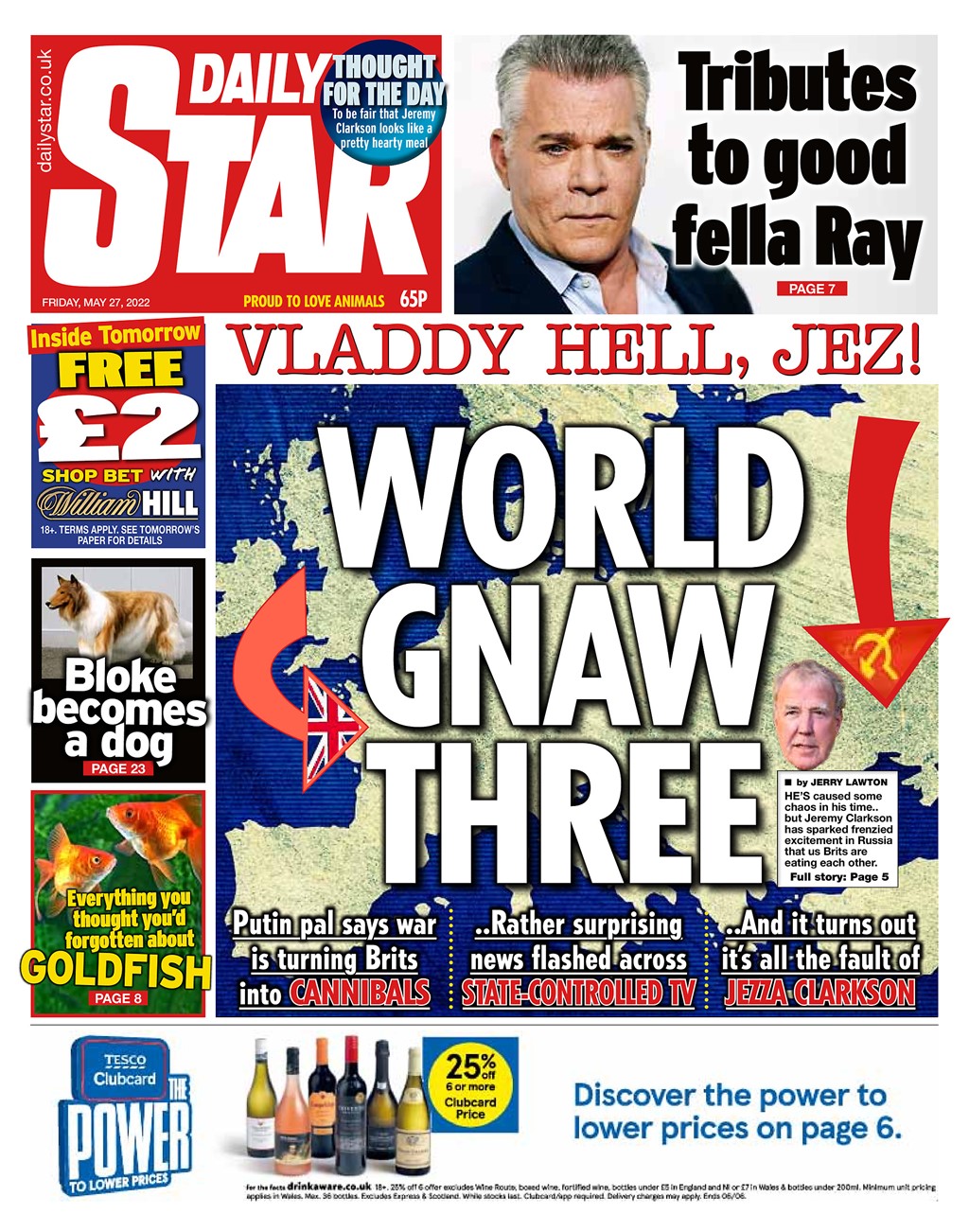The cover of the Daily Star magazine, dated Friday, May 27, 2022, is a collage of striking elements. 

In the upper left-hand corner, a red background hosts the white text "dailystar.co.uk," followed by the bold "Daily Star" title. Below it, the issue date "Friday, May 27, 2022" is inscribed, along with the price "65P." Next to this is a blue circle containing the white text "store for the day."

Jeremy Clarkson, described as a hardy male, makes an appearance, sparking frenzied excitement. A yellow banner declares "proud to love animals."

On the opposite side, the tribute to "Goodfellow Ray" is marked against a white background with black text. Adjacent is a red rectangle with the notice "page seven" in white text, referencing the actor from Goodfellas who played the main character.

Central to the cover, in bold red on a white background, reads "Vladdy Held, J, easy!" Overlaid on a stylized map featuring blue and yellow hues is the white text "world nod three." Below this, a politician’s face is paired with the byline "by Jeremy Lawton," hinting at the chaos caused by the individual.

A teaser for a full story on page five is marked by a red arrow with a yellow hook or axe and a Union Jack flag pointing downwards, drawing attention to the brewing situation involving Jeremy Clarkson and the frenzied excitement in Russia.